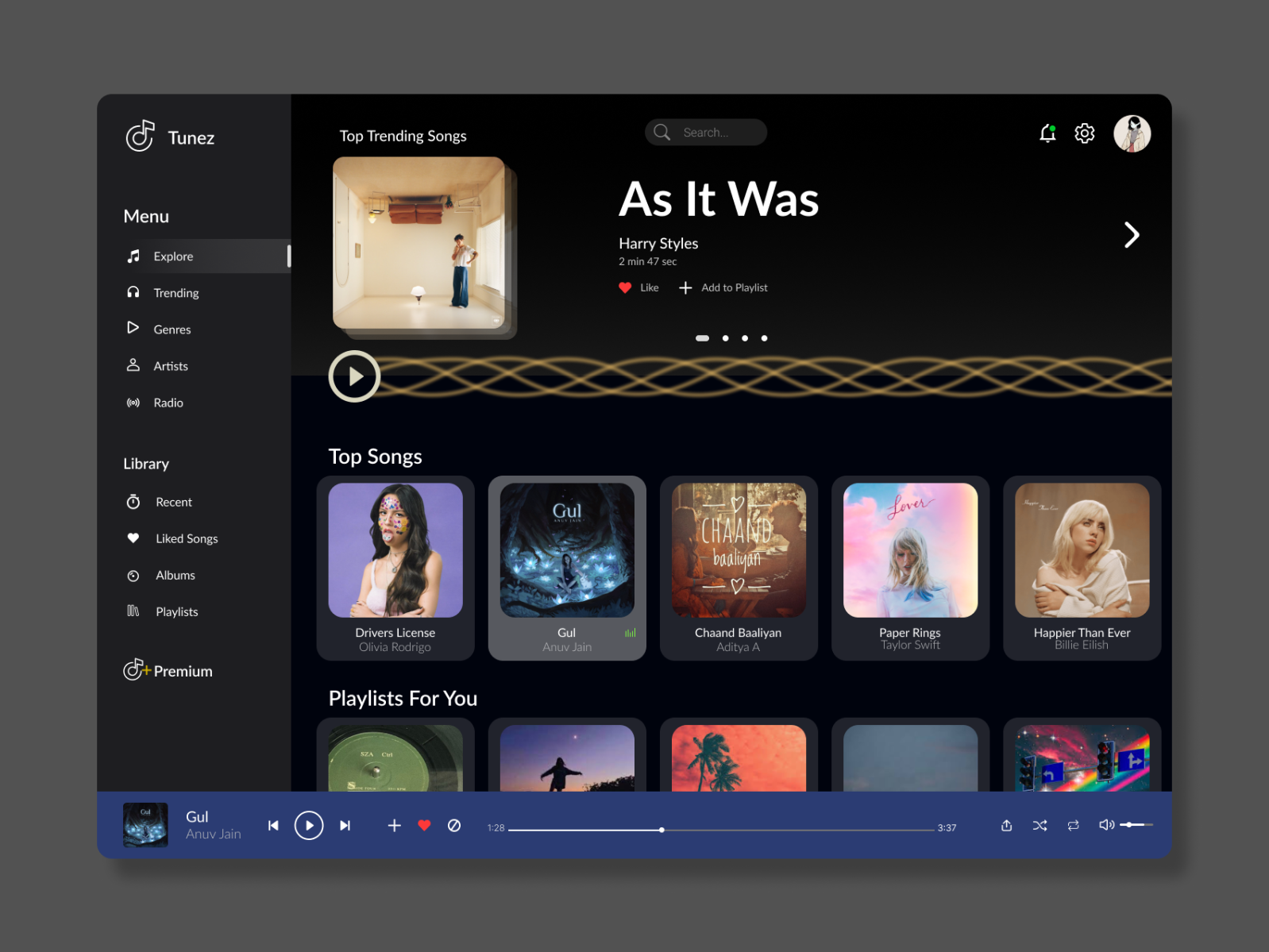This screenshot captures the sleek interface of a Tunes-type website. The background is a dark gray, which provides a modern and immersive feel. In the pop-up window on the left, there is a vertical menu. At the top, the header proudly displays the word "Tunes" in white, capitalized font accompanied by a music note logo, reinforcing the musical theme.

The vertical menu beneath the header organizes the site’s features. The main menu includes options such as "Explore," "Trending," "Genres," "Radio," and "Artists," all listed to guide users easily through the different sections of the site.

Below this primary navigation is the "Library" section, offering quick access to "Recent," "Liked Songs," "Albums," and "Playlists," catering to personalized content. Further down the menu, the word "Premium" indicates an area dedicated to premium services or content.

In the main content area of the site, there is a highlighted feature labeled "Top Trending Songs," featuring Harry Styles' "As It Was," which notably has a duration of 2 minutes and 47 seconds. Additionally, the screenshot includes thumbnails of other top songs, providing visual cues to popular tracks available on the platform.